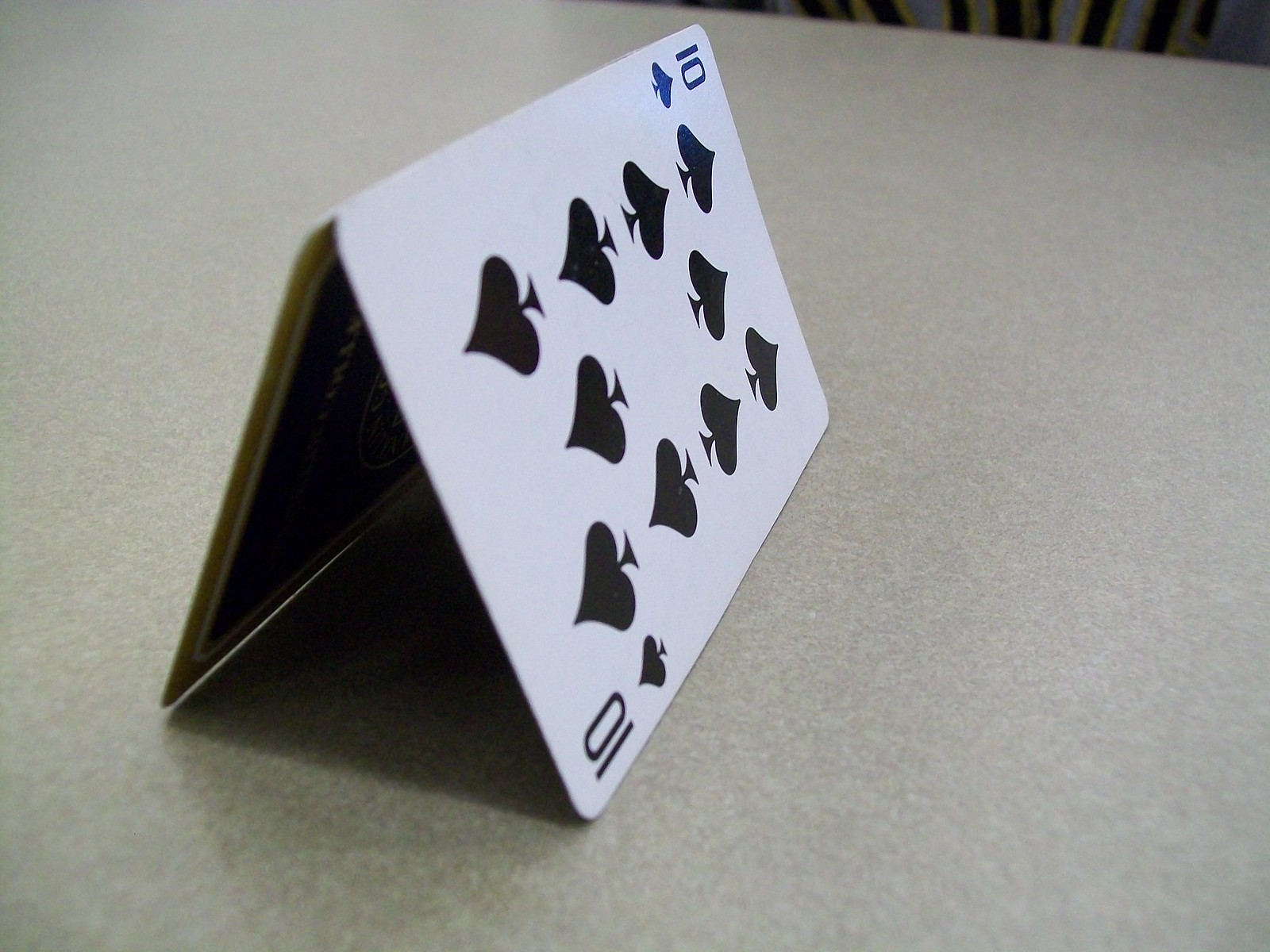In the photograph, two playing cards are strategically positioned on a table, creating a tent-like structure. The table surface is a gray Formica with a white, splotchy pattern, dominating the entire background except for the top right corner, which shows hints of black and white tones, likely beyond the table's edge. The two cards are almost the same height as the picture itself. 

The front card prominently displayed is the 10 of spades, impeccably clean with no smudges or marks. The 10 of spades symbol appears in the top left and bottom right corners of the card, nearly aligning with the top and bottom edges of the photo respectively. The second card, which supports the structure, reveals only its back. This card appears dark, possibly blue.

A distinct shadow is cast underneath the tent formed by the two cards, adding depth and realism to the image. The careful placement and detail in the photograph highlight the crisp, uncluttered state of the card and the interplay of light and shadow on an otherwise minimalist background.